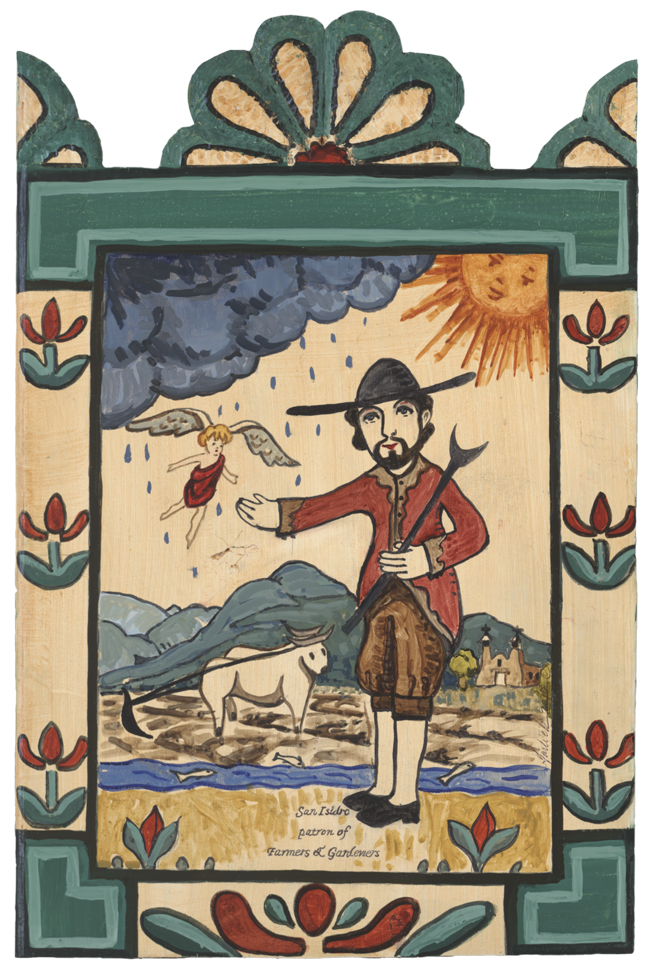This image depicts a detailed Spanish-style painting set against a tan background. At its center, there is a mural showcasing a historical farmer, who is likely San Ysidro, patron of farmers and gardeners, as indicated by the text. The farmer is dressed in a burgundy-colored jacket, brown knee-length pants, and black low-cut fur-like shoes. He wears a hat, which may be to shield himself from the sun or rain, and has dark facial hair.

The scene around him includes a variety of elements: a white animal, possibly a cow or an ox, appears in the background alongside vibrant flowers growing near the ground. The background stretches out to reveal distant mountains, with a Pueblo-style church visible far off. Above, the sky exhibits intricate details, with an angel flying down from rain clouds, and an orange sun with a smiling face looking down, contributing both sunlight and rain to the pastoral scene. Surrounding this central mural is a decorative flower pattern featuring dark green and red petals, completing the rich and symbolic artistry of the piece.